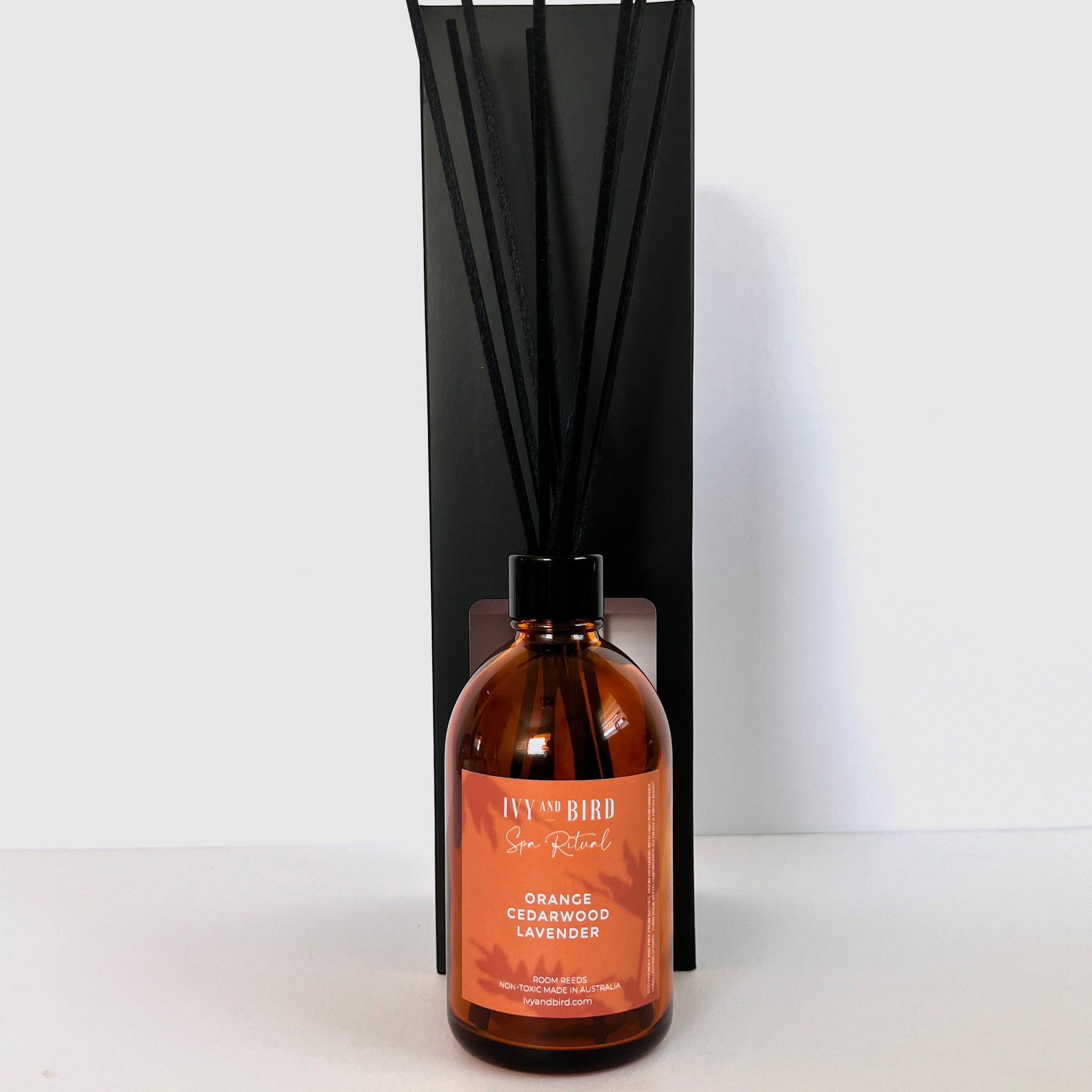This is an image showcasing a room fragrance diffuser. The focal point is a brown glass bottle with a sleek black top, through which several long black reeds extend to diffuse the scent into the surrounding area. The bottle is set on a white table against a white backdrop, with a tall black rectangular element directly behind it, possibly the packaging box, adding contrast to the composition.

The bottle features an orange label adorned with an abstract print of darker orange leaves. The label prominently displays the brand name "Ivy and Bird" and details the scent as "Orange, Cedarwood, Lavender." Additional information on the label notes that the product is non-toxic and made in Australia, with the website ivyandbird.com provided for further details.

The overall scene creates an elegant and minimalistic aesthetic, likely intended for promotional use, perhaps for a website advertisement. The white room and refined presentation enhance the appeal of the product, suggesting it as a sophisticated addition to any space for a pleasant aromatic experience.